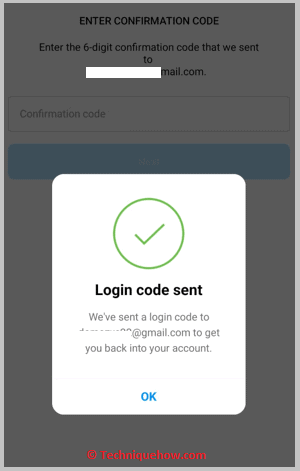A white square notification with a green circle containing a check mark in the center displays the message: "Login code sent." The notification informs the user that a login code has been sent to their email to assist in regaining access to their account. The website mentioned is TechnicianHowit.com, highlighting its role in facilitating the login process. The notification box stands out with its clean and straightforward design, ensuring users are clearly informed about the next step in the authentication process.